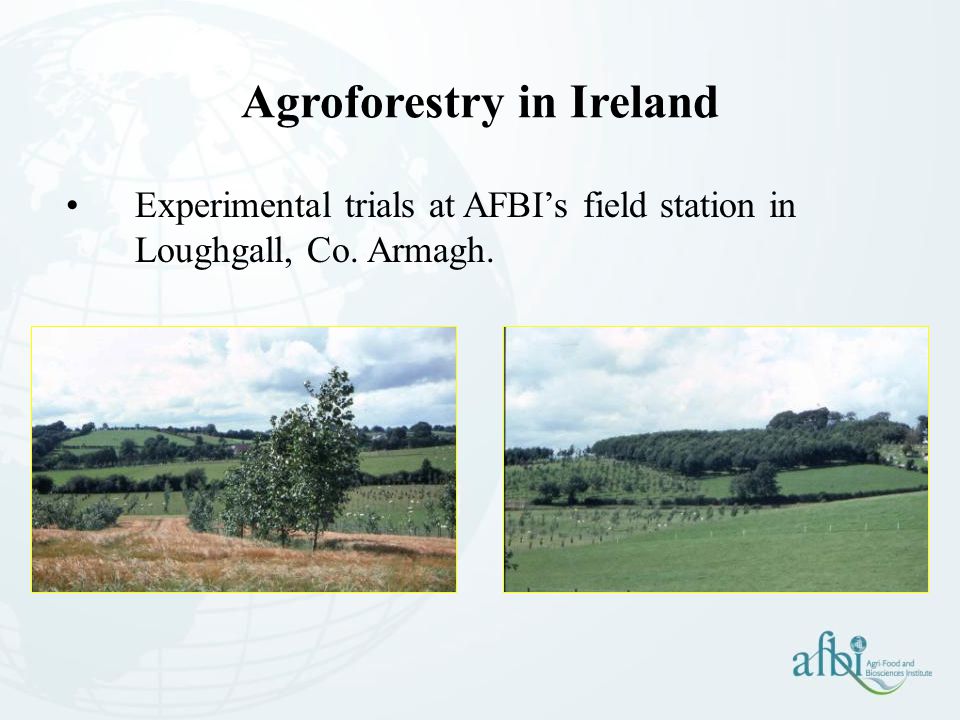The image titled "Agroforestry in Ireland" features two pictures showcasing AFBI's experimental trials at their Field Station in Loughgall, County Armagh. The header text is in bolded Times New Roman font, and a single bullet point underneath the title reads "Experimental Trials at AFBI's Field Station in Loughgall, Co. Armagh." There's an AFBI logo at the bottom right corner of the image.

The left picture shows a brown field with some trees in the middle. To the left of the trees are shorter bushes, while behind these trees stand two lines of darker green trees, separating the foreground from a large green field extending into the background. The sky is blue with many fluffy, white clouds.

The right picture depicts a large green field under a similarly blue and cloud-filled sky. In the top right corner of this field, there is a dense cluster of darker green plants, with a less dense area of smaller plants to its left. Both images prominently feature lush greenery and natural landscapes, emphasizing the agricultural and forestry aspects of the site.